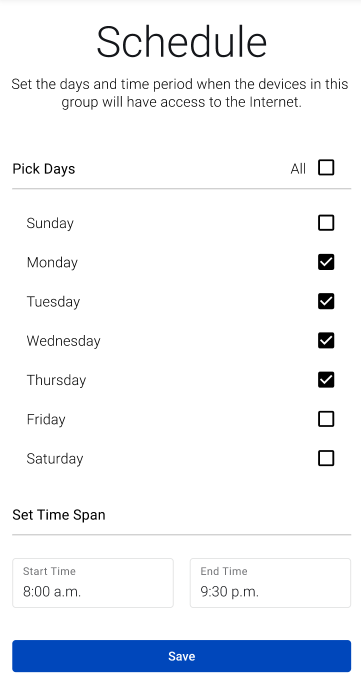The image appears to be a screenshot of a scheduler interface, with a clean, white background and all text rendered in black. At the very top, in a large font, the word "Schedule" is prominently displayed. Directly below, in smaller text, it instructs the user to "Set the days and time period when the devices in this group will have access to the internet."

There is a section titled "Pick Days" on the left, accompanied by an "All" checkbox on the right, which can be selected to apply the settings to every day of the week. A thin line separates this option from a list of individual days, starting from Sunday and ending on Saturday, each with its own clickable checkbox. Currently, Monday, Tuesday, Wednesday, and Thursday are checked, indicated by a filled black box with a white checkmark.

Below this section, to the left, is the heading "Set Time Span," followed by another divider bar. Here, the schedule can be further customized with start and end times. A box labeled "Start Time" indicates the devices will begin accessing the internet at 8:00 AM, and to its right, an "End Time" setting shows access will cease at 9:30 PM.

At the very bottom of the interface, a blue rectangular bar displays the word "Save" in white font, which finalizes the settings. The entire interface appears devoid of any additional overlays, notifications, or visual distractions, ensuring the user's focus remains on configuring the scheduler.

This scheduler allows for precise customization of internet access, evidenced by the detailed daily and hourly configuration options and the clean, user-friendly design aimed at simplifying the process.